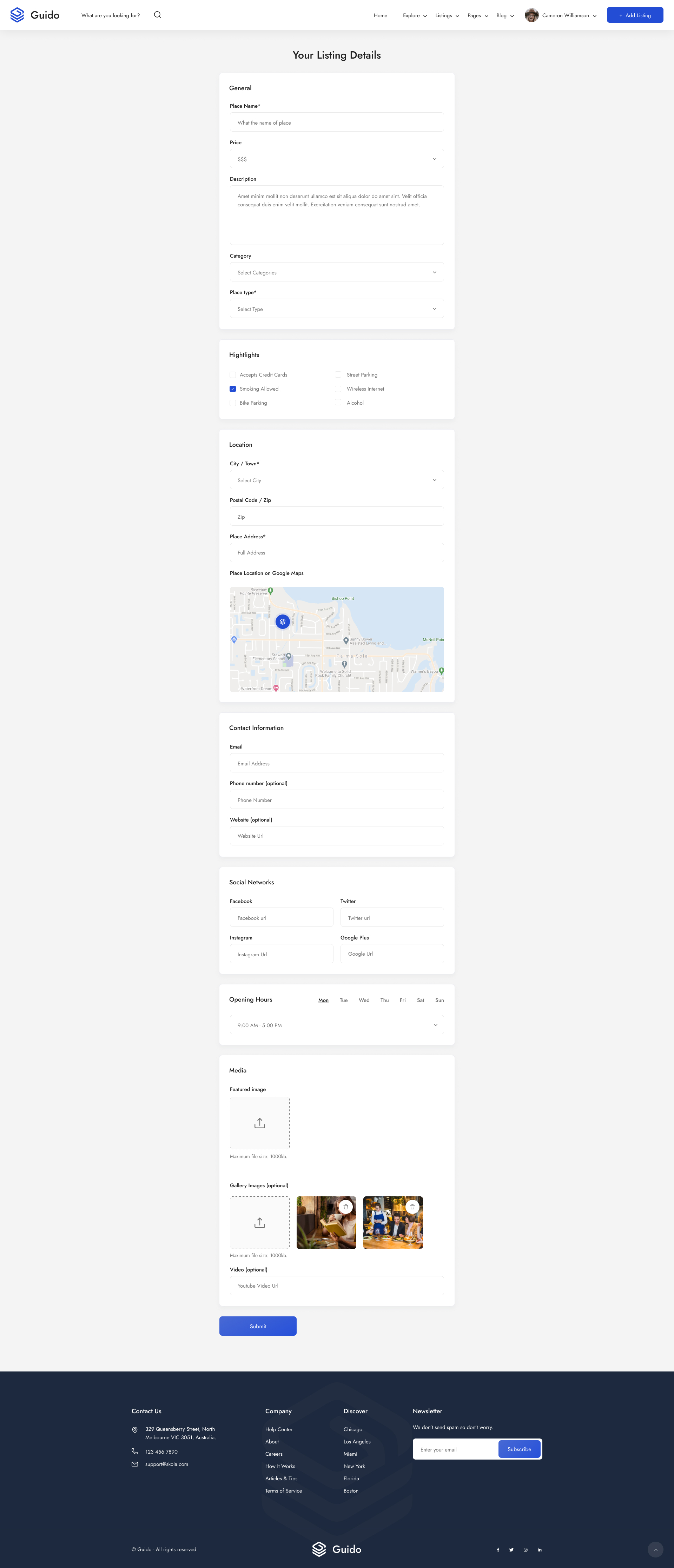This detailed caption succinctly describes the elements visible in the image:

---

The image showcases a modern webpage designed to guide users through listing details. At the top of the page, "Guide Your Listing Details" is boldly written in black letters against a clean white background. Below this title is a photo of a map reminiscent of Google Maps, adding a geographical context. At the bottom of this map, there are two photos side by side, giving additional visual content. Adjacent to these images, a gray square with an upward arrow symbol indicates an upload area, suggesting that users can upload their own images or documents.

Towards the bottom of the page, there's a distinct blue button for user interaction. Directly above this button, the interface provides options such as "Contact Us," "Company," "Discounts," and "Newsletter." To the right, a white box prompts users to enter their email for subscription, with a blue button labeled "Subscribe" in white letters. The overall background of the page is predominantly gray on the edges with a white center, and the footer has a contrasting black background. At the top right corner, there is another blue button, complementing the blue "Subscribe" button. The logo, positioned next to "Guide Your Listing Details," features three stacked squares with the letters "GUIDO."

---

This caption not only describes the visual elements but also contextualizes their functionality and layout, providing a comprehensive overview of the webpage's design.